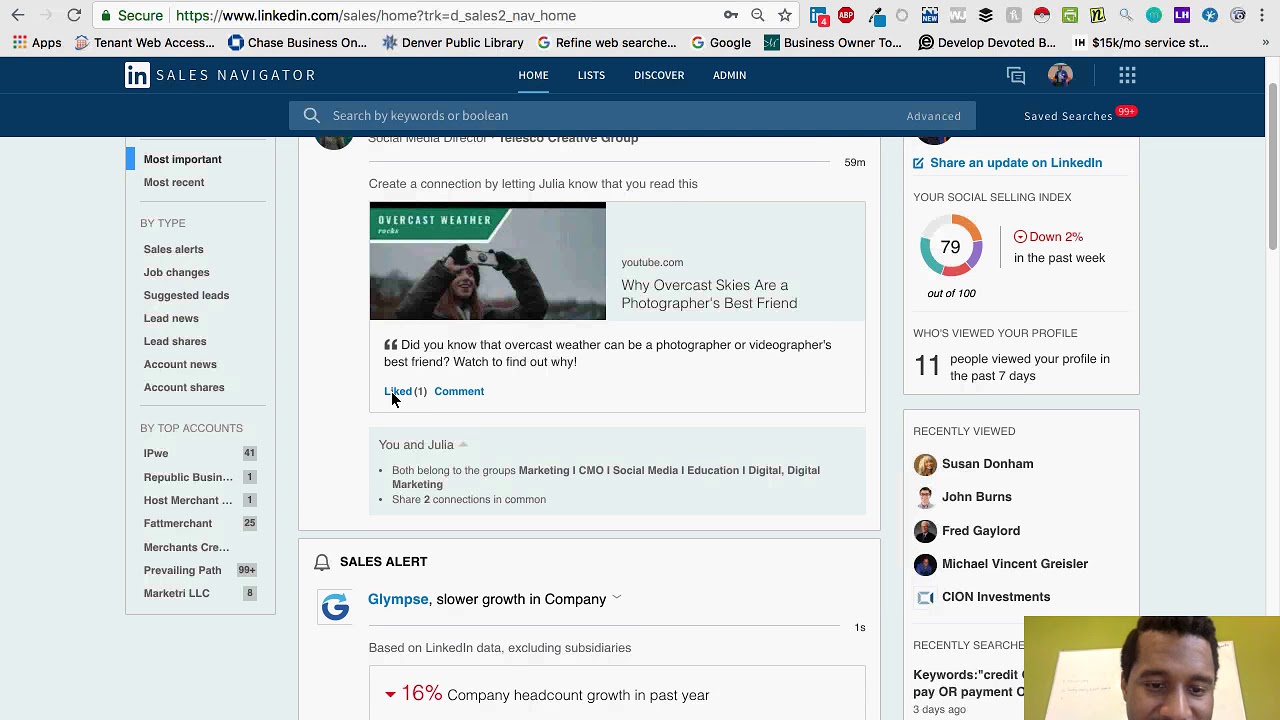Screenshot of a cluttered desktop interface showing a LinkedIn Sales Navigator webpage. The URL is visible at the top, indicating LinkedIn as the website. The user is on the Sales Navigator homepage, which displays an abundance of data and compact text. At the top of the page, it reads "InSalesNavigator," confirming it as a navigational tool for sales professionals. The user's bookmarks bar is unusually crowded with numerous shortcuts and applications, reminiscent of an unorganized desktop.

On the right side of the LinkedIn page, several widgets are prominently displayed. One widget shows the user's Social Selling Index (SSI), which stands at 79 out of 100, noting a 2% decrease over the past week. Another widget lists profile view statistics, indicating that 11 people have viewed the user’s profile in the last 7 days. Below this is a section for recently viewed accounts, displaying names such as John Burns and Fred Gaylord.

The overall impression is one of a busy, information-dense interface with numerous features competing for attention.